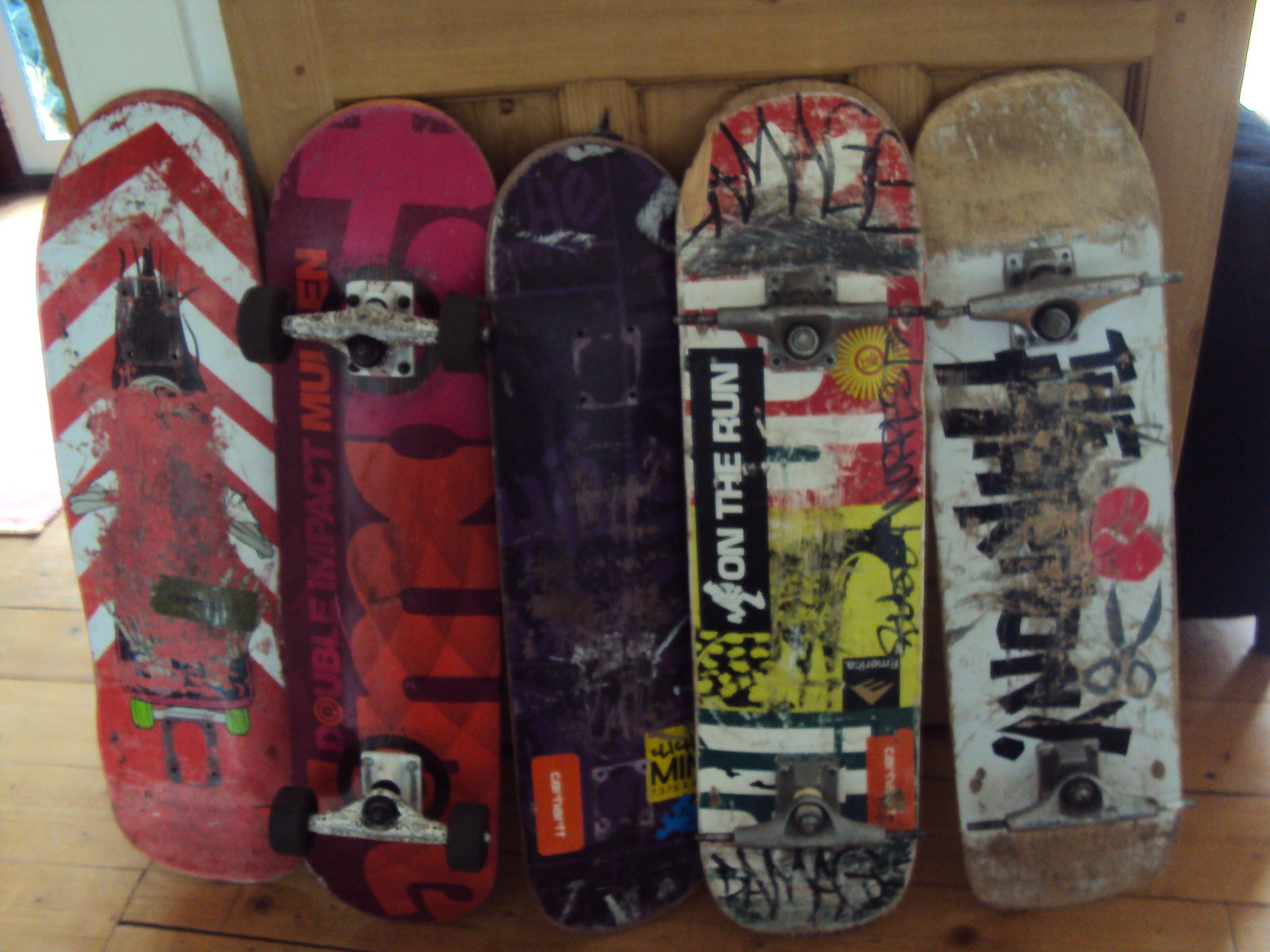A detailed photograph depicts five heavily worn skateboards propped vertically against a wall, resting on a light tan oak hardwood floor characterized by small gaps between the panels. The backdrop includes a white wall and a light brown wooden door, possibly indicating an entrance. In the vicinity, a blue sofa adds color to the indoor scene.

1. The skateboard on the far left lacks wheels and features a deteriorated design with red and white chevrons, showcasing a chipped and faded drawing obscured by red paint.
2. Adjacent to it, the second skateboard, adorned with red coloring and intricate orange and red diamond patterns, includes the text "Double Impact" and has its spokes but no wheels.
3. The middle skateboard stands out with its dark coloration, marked by scuffs and damage. It does not have wheels or spokes but possesses red and yellow labels.
4. The fourth skateboard has two spokes but no wheels, and its surface is scribbled with various black marker writings, black and yellow designs, and a distinctive "On the Run" sticker.
5. The skateboard on the right is the most damaged, with both ends sanded to reveal the bare wood. The center, painted white, is chipped and features a fading red heart with scissors and some largely indecipherable black text.

The skateboards, differing in color and design but unified by their visible wear and tear, tell a story of usage and history.